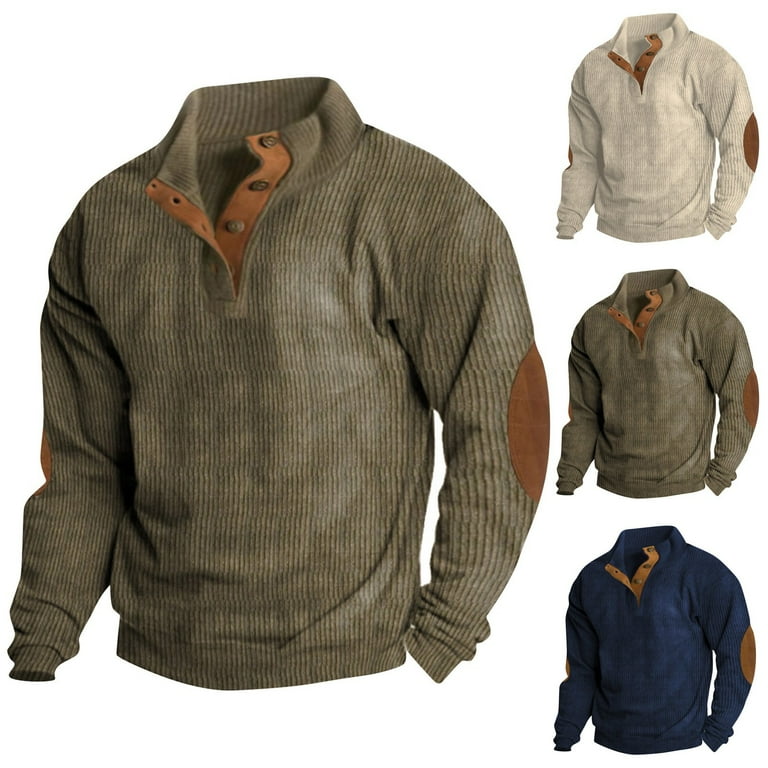This advertisement image features a collection of men’s pullover sweaters meticulously displayed against a white background. The sweaters showcase a distinctive rib knit texture reminiscent of corduroy and come in various colors: olive green, beige, brown, and navy blue. Each sweater is adorned with dark brown leather patches on the elbows and a leather strip around the collar with matching buttons, providing a rugged yet sophisticated look. The advertisement displays one of the sweaters, the olive green one, in both a standard and an enlarged view for detailed inspection, emphasizing its intricate material and design. The consistency in detailing across all sweaters, where only the primary colors vary, creates a cohesive and appealing presentation for potential buyers.